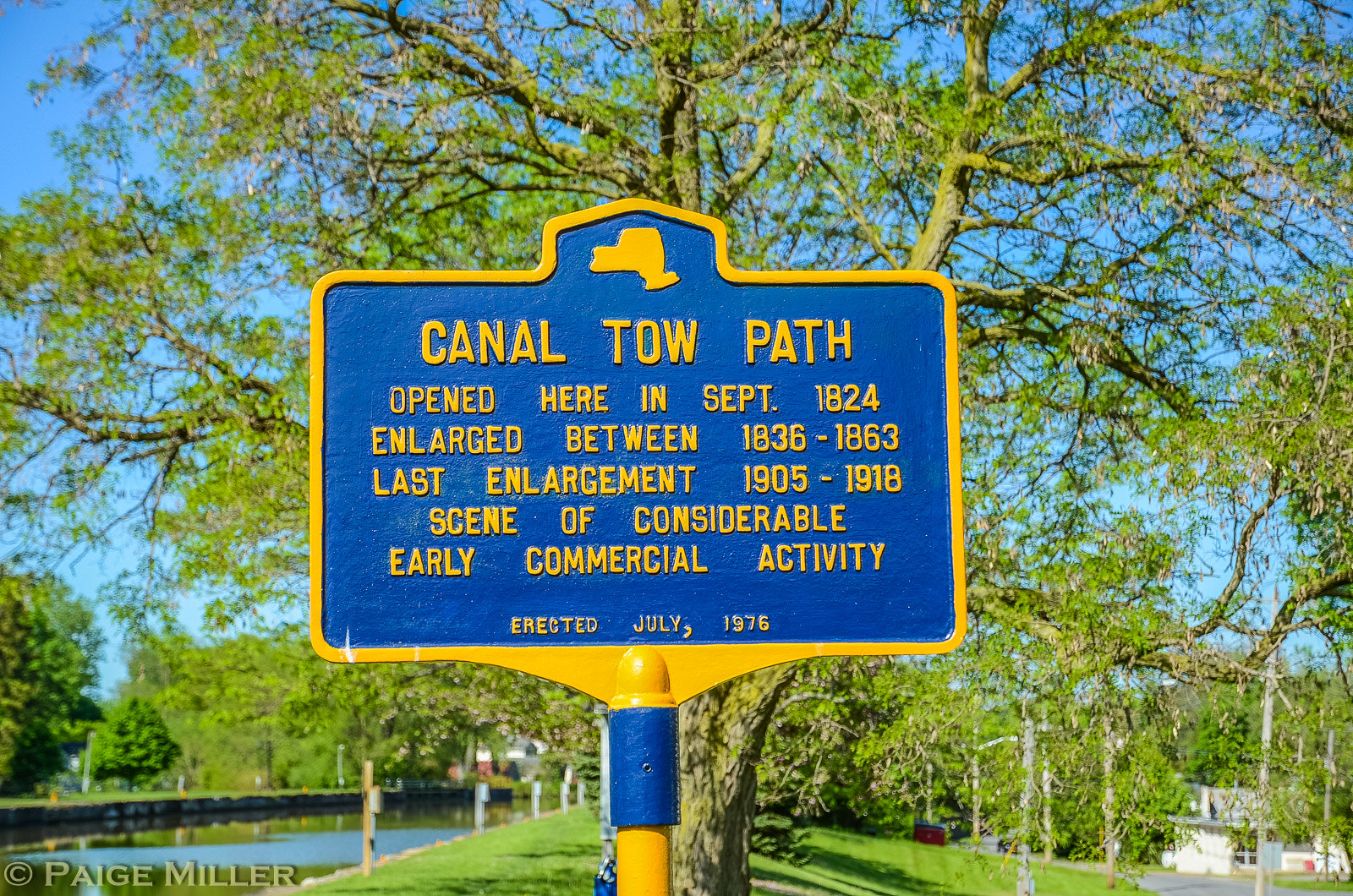In this vibrant park scene, an upright sign prominently stands out, characterized by its distinctive blue background with a fluorescent yellow border and text. The sign, featuring the symbol of a simplistic house at the top, reads "Canal Towpath" and provides a historical timeline: opened in September 1824, enlarged between 1836 and 1863, and further expanded from 1905 to 1918. Beneath this informative text, it notes the sign was erected in July 1976. A notable yellow pole supports the sign, which extends out of view at the bottom. The park itself is lush with green grass and dotted with large trees full of vibrant green leaves. A strip of water, likely a lake or river with a brownish-blue hue, runs alongside the greenery. The scene is illuminated by bright daytime light, under clear blue skies, creating a peaceful and inviting atmosphere. In the bottom left corner of the image, a light gray watermark reads "Page Miller," accompanied by a C trademark icon. The entire setting is free of any human presence, emphasizing a tranquil, natural environment.